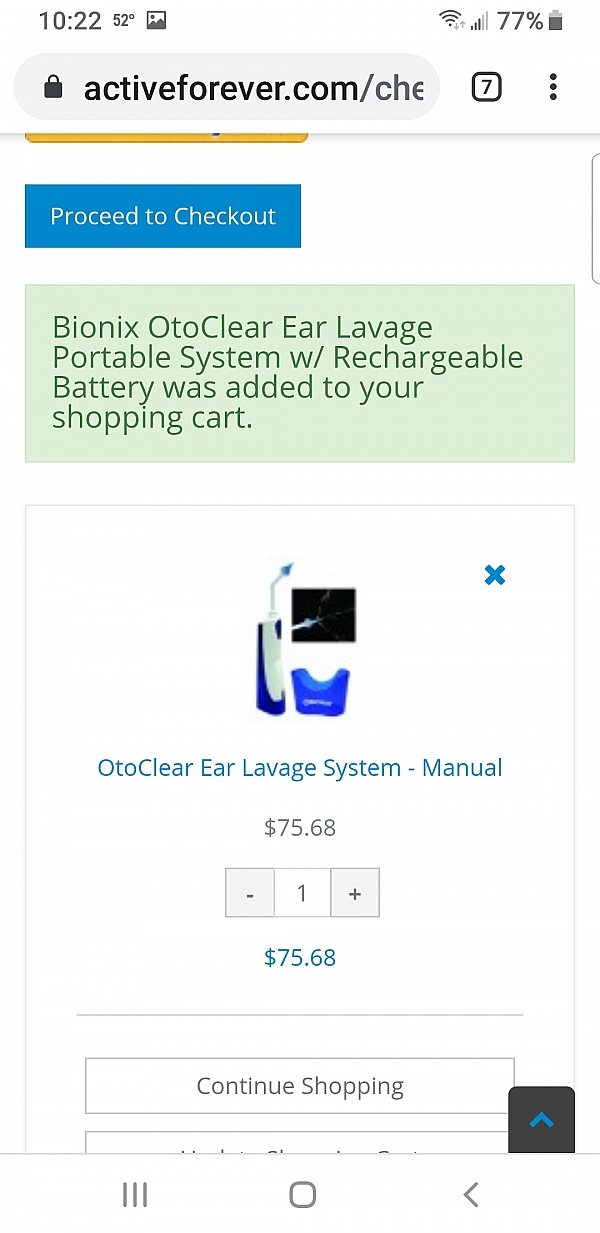A screenshot of a cell phone displaying a web page. The device's status bar at the top shows the time as 10:22 AM on the left, alongside a temperature reading of 52 degrees and a picture icon. On the right side, the Wi-Fi signal strength is indicated at 77%, next to the battery icon. Below the status bar, the web address indicates the user is on the checkout page of ActiveForever.com.

The main content of the screenshot shows two prominent buttons: a blue rectangle saying "Proceed to Checkout" in white text, and a larger green rectangle that reads "Bionix Otoclear Ear Lavage Portable System w/ Rechargeable Battery was added to your shopping cart" in dark green text.

Beneath this, the page displays an image of the product, which resembles a water floss pick with a blue container holder next to it. Further details about the product include the name "Otoclear Ear Lavage System Manual" and the price listed as $75.68. There are buttons to adjust the quantity, and the price is reiterated at $75.68 in blue text below.

At the bottom of the screenshot, a white rectangle with black text provides the option to "Continue Shopping."